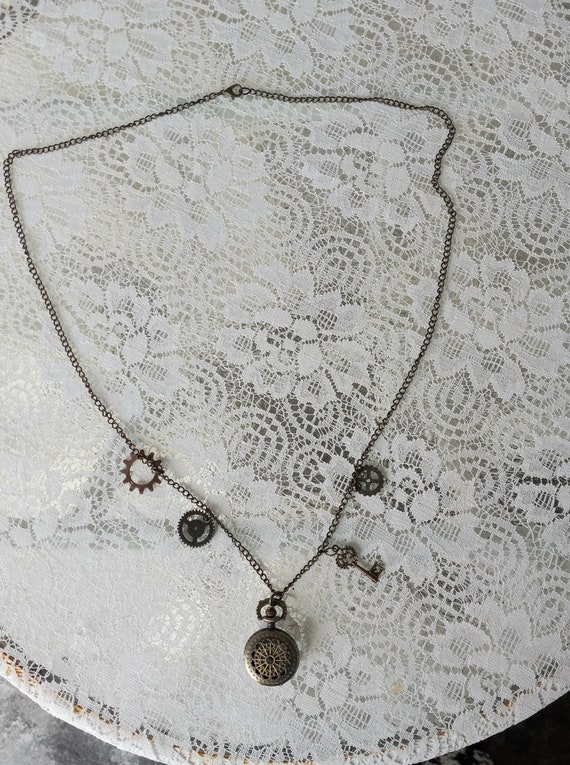This captivating photograph showcases an antique charm necklace artfully laid out on a white lace doily, which is displayed in an embroidery hoop. The image, taken from a top-down perspective, captures the intricate details of the necklace and its surroundings. The doily, presumably resting on an unseen table, provides an elegant and delicate backdrop for the aged necklace.

The necklace itself, composed of a dark-colored chain that could be tarnished silver or copper, features several charms that exude an old-fashioned aesthetic. The primary charm is a locket designed to resemble a vintage compass. Accompanying it are smaller charms, including an old-fashioned key and multiple gears, adding to its steampunk vibe. The photograph is rendered in black and white, enhancing the antique and timeless feel of the composition, with a focus on the texture and form of both the lace and the necklace.